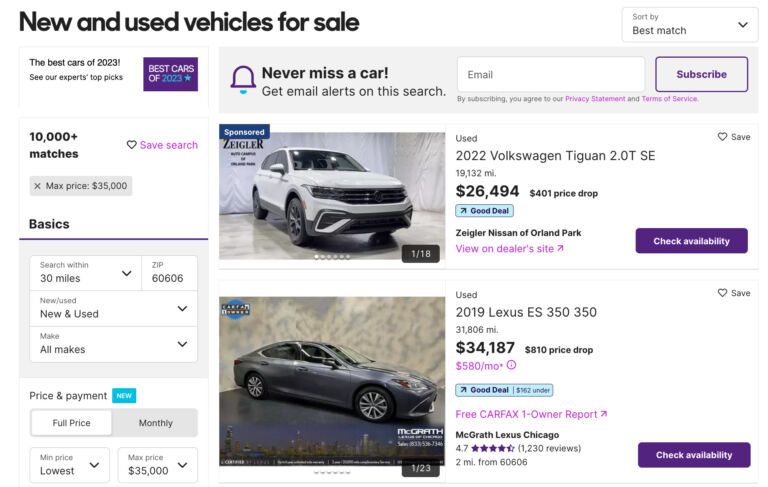**Detailed Caption:**

A user is exploring a car buying and sale website that offers a range of new and used vehicles. At the top of the page, a banner states "New and Used Vehicles for Sale," and the user is currently sorting the listings by "Best Match." The left side of the screen highlights the "Best Cars of 2023" along with links to expert topics and reviews. Adjacent to this is a banner featuring a small purple bell icon, with the prompt "Never miss a car, get email alerts on this search," offering users the option to subscribe to email notifications.

The search results reveal over 10,000 matches for the user's criteria, with a maximum price limit of $35,000. The search is filtered to show cars within a 30-mile radius of the 60606 zip code and includes various makes and models.

Two highlighted options catch the user's attention:

1. **2022 Volkswagen Tiguan 2.0 TSE**: Priced at $26,494, which is a $401 price drop. This vehicle, available at Ziegler Nissan of Orland Park, has 19,132 miles on it and is noted as a good deal. Users can visit the dealer's site for more information.

2. **2019 Lexus ES 350**: This car is listed at $34,187, featuring a significant $810 price drop. It has 31,806 miles on it, with an estimated monthly payment of $580. Details about the loan duration are not provided. The Lexus is also marked as a good deal, and users can access the owner's report through the website.

The user interface is neatly organized to facilitate an efficient and comprehensive car shopping experience.